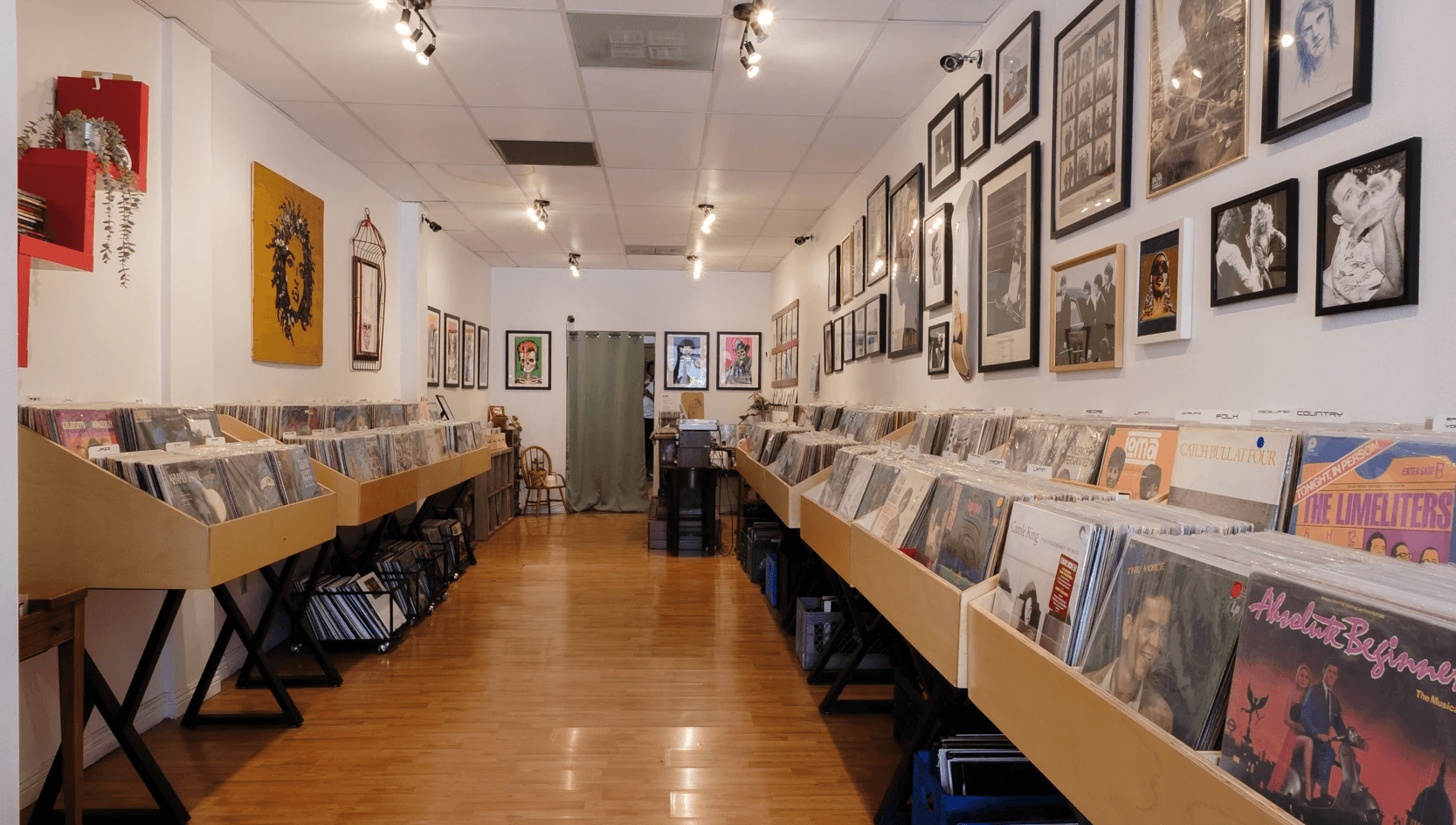This photo captures the interior of a cozy, narrow record shop, approximately 15 feet wide and 30 feet deep. The shop features an old, shiny brown floor that leads you through rows of meticulously arranged records. On the left side, there are three to four display cases made of tan wood with dark brown legs, each holding about 50 records in three rows. The right side showcases four display cases also with three rows of around 50 records each. Underneath these display racks, black wire bins offer additional records. The walls are adorned with an array of framed photographs and posters, all in black frames, featuring musicians, Hollywood characters, and various artworks. Dominating the back wall is a sage green curtain, suggesting an entryway into a backroom. Track lighting illuminates the scene, highlighting a rectangular mustard yellow canvas with a woman's face among the other eclectic décor elements scattered throughout the store.